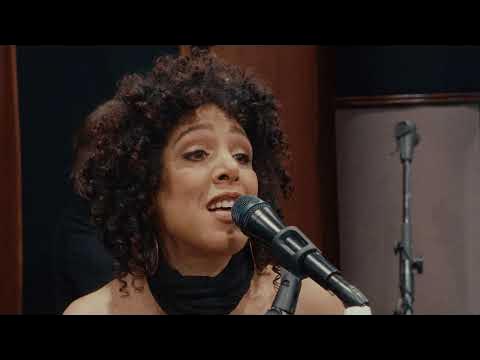The image captures a Latina or African American woman with dark, kinky, or curly hair, styled in a voluminous and somewhat afro-like manner, singing intently into a black microphone. She has light skin and is dressed in a black scarf or turtleneck, with what might be a guitar strap around her shoulder. The background features dark wood paneling in shades of black and brown. To her right, there is an unused microphone on a stand. The image, possibly a screenshot from a music video or television show, includes white screen bars indicating it's likely from a video format. The setting appears to be a studio or a similar indoor environment. The woman's focused gaze and the specific setting suggest she might be recording or performing, possibly identified as singer Raya Yarbrough.